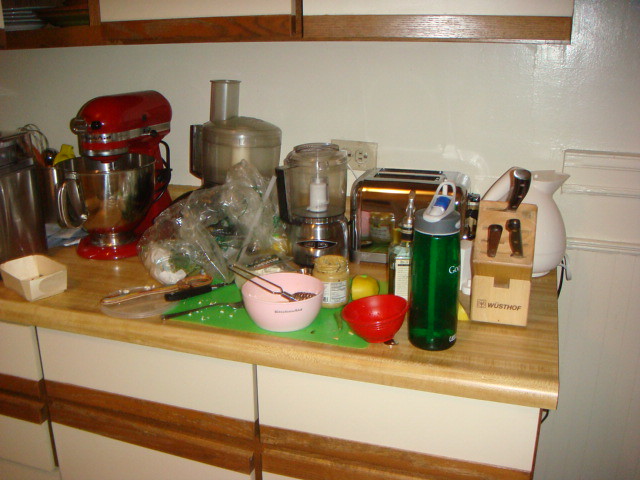The image depicts a cluttered kitchen counter showcasing an array of appliances and utensils, meticulously organized yet appearing busy. On the far left, a stainless steel vessel stands upright, filled with a whisk and other cooking implements. Beside it, a vibrant red stand mixer with a stainless steel bowl dominates its surroundings. Just in front of the mixer, there is an open white container.

Adjacent to the stand mixer, only the top part of a food processor is visible, revealing the hopper and feed tube. A plastic bag lies in front of it, contents indiscernible. Next in line is a smaller food processor with a sleek stainless steel base, followed by a practical two-slot toaster. Further to the right, a white pitcher completes the lineup of appliances along the back wall.

In the foreground, several items clutter the counter's surface. White bowls, possibly holding a spoon or tea infuser, a small red bowl, and a green water bottle with a grey top are scattered among various knives and spoons. The counter itself is a builder-grade butcher block, providing a warm, rustic feel that contrasts sharply with the tan colored cabinets below. These cabinets are designed with a unique molding at the bottom, providing a groove for easy opening, thus eliminating the need for knobs, and feature a dark wood finish on the groove, adding a touch of elegance to their functional design.